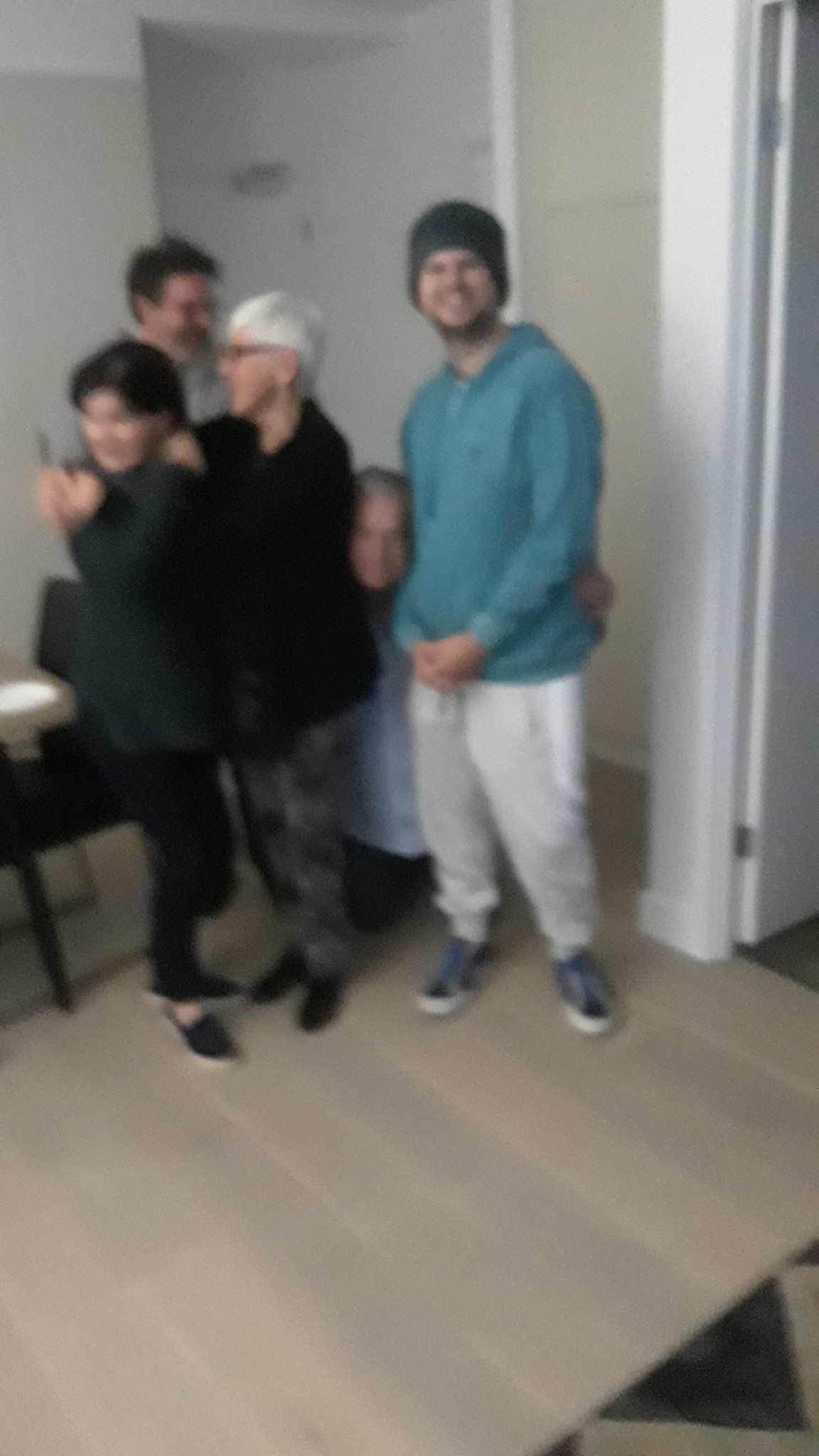The image is a family photograph, albeit very blurry, making it difficult to discern specific details. There are five individuals depicted, positioned from right to left. 

On the right-hand side, a man stands wearing a beanie, a bluish hoodie, white slacks, and predominantly black and white tennis shoes, with traces of blue visible. Next to him, a person with gray hair kneels on the ground, dressed in a baby blue button-up shirt and black slacks. This kneeling individual has an arm around the man in the blue hoodie and possibly extends it to embrace others, although the hand is not clearly visible.

To the left of the kneeling figure are three more people. The first of these is someone with short white hair and glasses, wearing a black jacket, gray or gray camo pants, and black footwear. This individual is hugging a woman with black hair, who is gazing towards the left side of the photo. She is dressed in a dark gray long-sleeved shirt, dark pants—either black or blue—and black slip-on shoes. Behind this embracing pair stands another man with brown or black hair, sporting a gray hoodie. 

The family appears to be standing in a hallway, with a white door visible on the far right and a cream-colored background suggesting an entryway or an adjacent hallway. A table is noticeable in the background to the left of the image, adding to the sense of a homely environment.